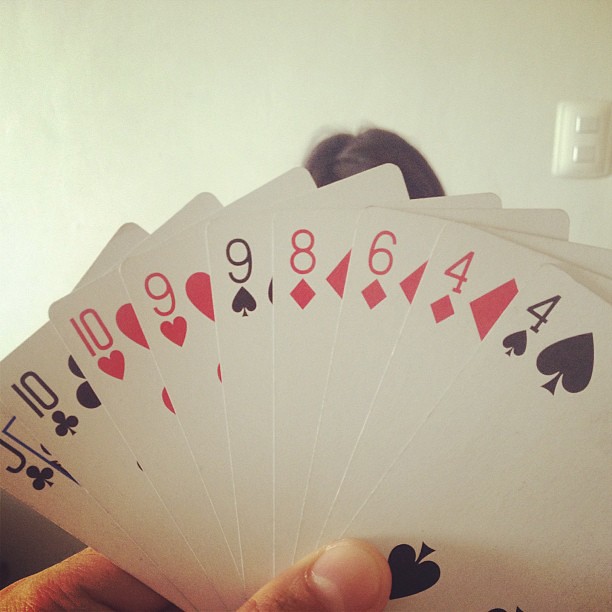An up-close photograph captures a hand of playing cards held by an indistinct player. The cards are fanned out, revealing a sequence from left to right: the Jack and Ten of Clubs, the Ten and Nine of Hearts, the Nine of Spades, the Eight, Six, and Four of Diamonds, and the Four of Spades. The thumb and the base of the index finger are visibly gripping the cards. In the background, the faint outline of another player's hair is visible over the top of the cards, against a stark white wall. A light dial used to control the room's lighting is also seen on the wall. Natural daylight streams in from the left, suggesting the presence of an open window outside the frame, illuminating the scene and indicating daytime. This detailed arrangement and lighting evoke a casual yet focused moment in a game, possibly rummy, as evidenced by the ordered suits and numbers on the cards.